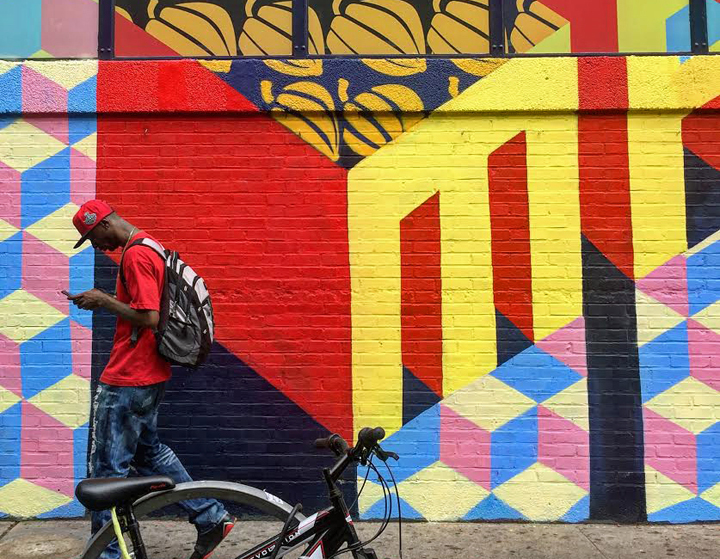The horizontal rectangular image features a vibrant, mural-painted brick wall with abstract and geometric designs in vivid colors like pink, blue, yellow, and red. A young African American man, wearing a red t-shirt, blue jeans, red baseball cap, backpack, and a necklace, walks along a sidewalk from right to left. He is looking down at his phone, which he holds with both hands. In the foreground, closer to the camera than the sidewalk, a dark-colored bicycle is locked to a bike stand. The wall beside him showcases a mix of disparate abstract art, including alternating pink, blue, and yellow blocks, alongside three-dimensional yellow letters that appear angled, possibly forming a compact shape resembling a "V" or "E." Above this, a pattern reminiscent of blue and golden pumpkins or bananas adds to the vivid visual appeal. The entire mural provides a colorful and dynamic backdrop to the everyday scene of the man engrossed in his phone on a city street.